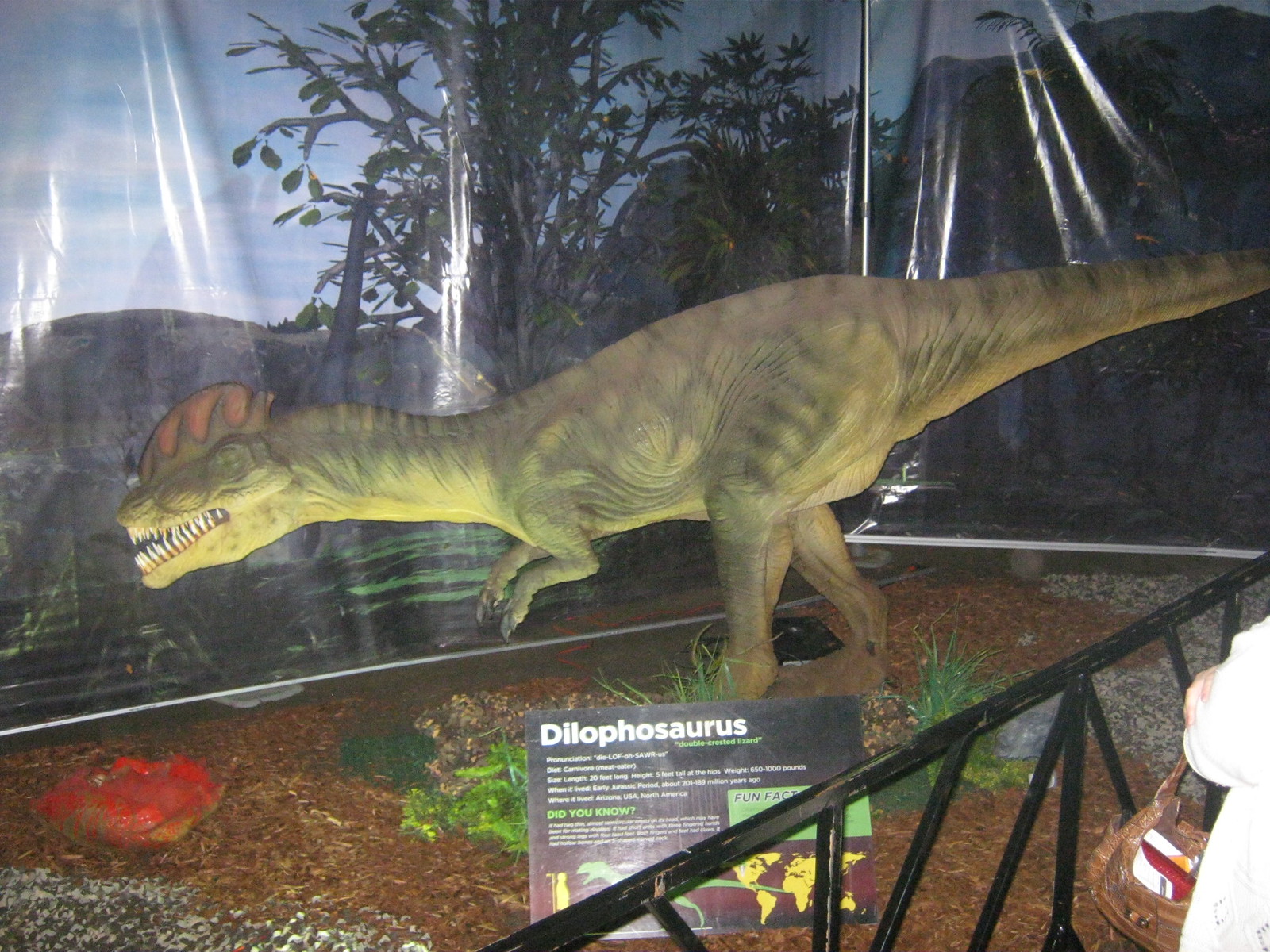The image is a detailed photograph taken inside a historical or science museum. It captures a meticulously crafted diorama showcasing a life-sized model of a Dilophosaurus. The dinosaur model, predominantly green with grayish stripes, brandishes sharp white teeth and a distinctive green and red crest on its head. It stands on two hind legs, leaning forward with its raised tail, displaying a dynamic and lifelike posture.

The base of the display is covered in a brown mulch-like substance, adorned with small green plants and what appears to be a red representation of a prey it has hunted. This foundation is designed to mimic the earth's surface as it would have appeared during the dinosaur's era. 

In the foreground, a black metal barrier runs diagonally from the midline to the upper right-hand corner, preventing visitors from entering the display area. The lower right corner of the photograph captures a person's arm holding a brown bag, suggesting they are engaged with the exhibit.

An informative black rectangular sign is positioned prominently at the base of the dinosaur model. The sign features white lettering that reads "Dilophosaurus," with a subtitle in green, "double-crested lizard." It includes detailed information on the dinosaur's pronunciation, diet, size, period of existence, and interesting facts. An illustration on the sign compares the dinosaur's size to a human male, indicating that a full six-foot-tall human would stand at the level of the dinosaur's mouth.

The backdrop of the diorama is a plastic screen depicting a vibrant scene of tall trees, large rock cliffs, and a clear blue sky, enhancing the realism of the display. Overall, the diorama offers an immersive and educational glimpse into the prehistoric world of the Dilophosaurus.